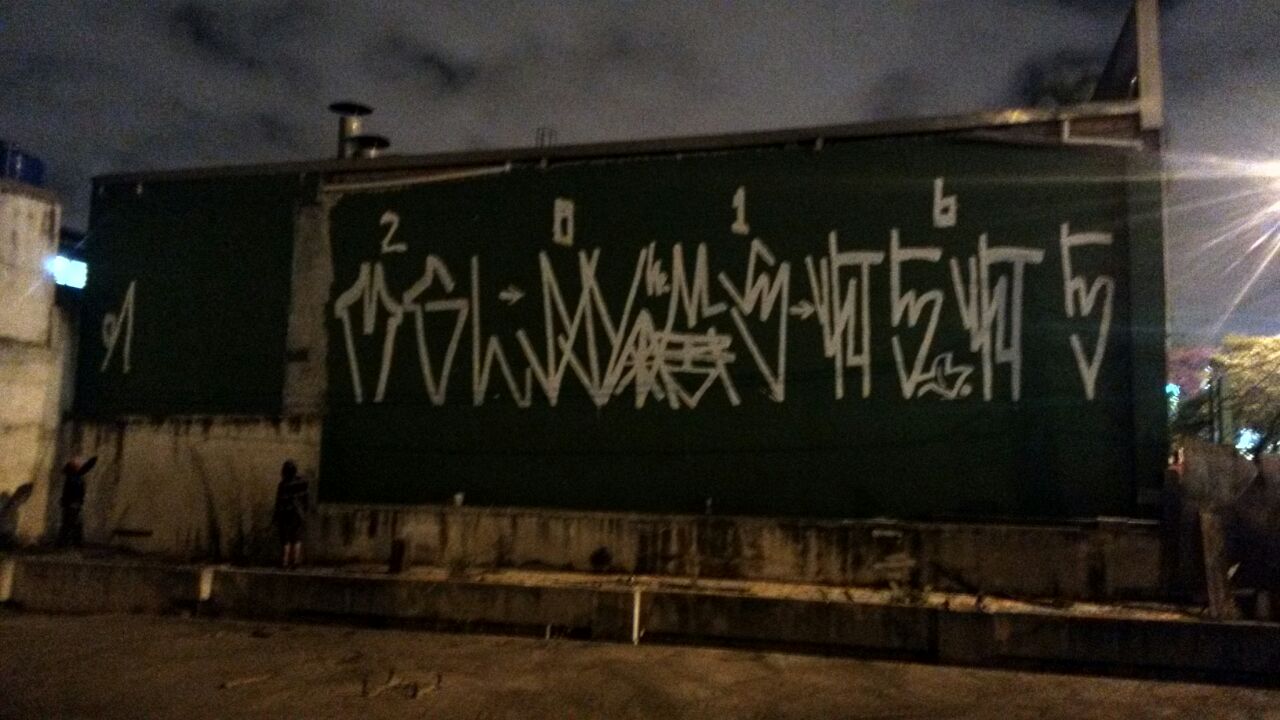The image captures a night scene outside a dilapidated building with a graffiti-covered wall. The predominant feature is a large banner mounted on the grey, grimy surface of the wall. The banner showcases the numbers "2016" prominently at the top in white lettering against a green background, followed by an array of unconventional, unreadable symbols spanning its width. To the left, a second banner displays just a single upside-down V symbol. The scene is lit by lights from either side, possibly street lamps, casting their beams onto the area. The surroundings are stark and neglected, with a grey cement ground and a step leading up to the wall. Two people are present in the background – one gazing up at the banner, while the other reaches towards the hanging section of the second banner. The dark, cloudy night sky looms above, adding to the desolate atmosphere.